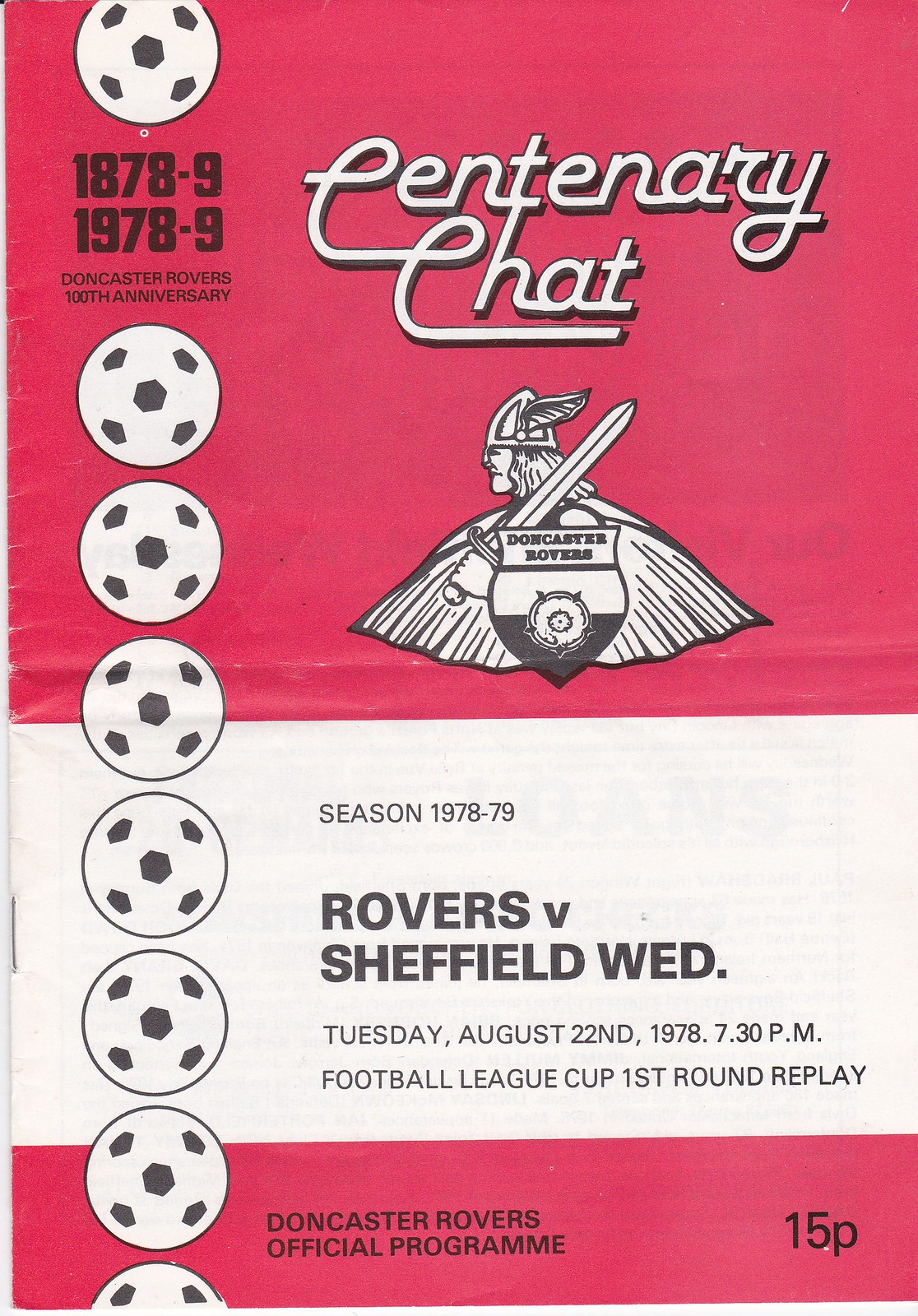The image is a detailed vintage soccer program cover for the Doncaster Rovers' 1978-79 season, commemorating their 100th anniversary. The background is a reddish-pink color with a striking white stripe at the bottom. At the top, the headline reads "Centenary Chat," followed by a prominent illustration of the Doncaster Rovers' Viking mascot holding a sword and shield. On the left side, a vertical column features eight football images, with annotations marking the years 1878-9 and 1978-9 to emphasize the centenary celebration. Below the mascot, in the white section, the text highlights the "Rovers vs. Sheffield Wednesday" match scheduled for Tuesday, August 22, 1978, at 7:30 p.m., as a Football League Cup first round replay. The program is priced at 15p, and at the bottom in the pink stripe, it reads "Doncaster Rovers Official Program," marking this as an official piece of memorabilia.